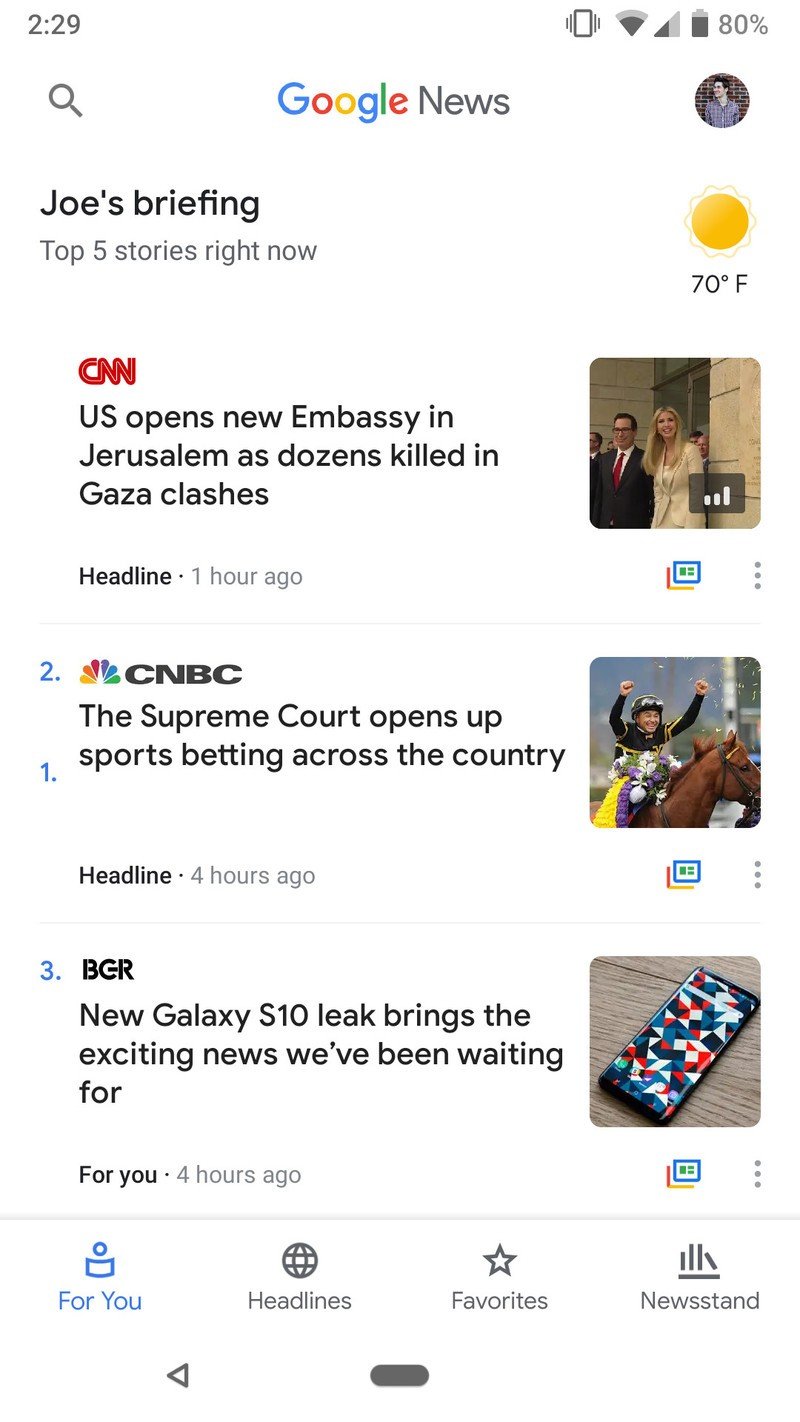This image is a screenshot of a Google News feed taken at 2:29. The top status bar indicates a strong Wi-Fi connection and an 80% battery level. On the top left, there is a magnifying glass icon just beneath the time. The Google logo is displayed in its standard multicolored font next to the word "News" in dark gray. To the right, the user's profile picture is visible.

Beneath the heading, the text "Joe's briefing" is written in black font, followed by "Top five stories right now" in a lighter gray font. To the right of these headings, it indicates a sunny weather with a temperature of 70 degrees Fahrenheit.

The feed begins with a story from CNN, identifiable by the red CNN logo. The headline reads, "U.S. opens new embassy in Jerusalem as dozens killed in Gaza clashes," and is marked as being posted one hour ago. There is an option for audio playback associated with this article.

The next story, from CNBC, features their recognizable multicolored peacock logo. The headline states, "The Supreme Court opens up sports betting across the country."

The third visible story originates from BGR, though the headline content is not provided in the given text.